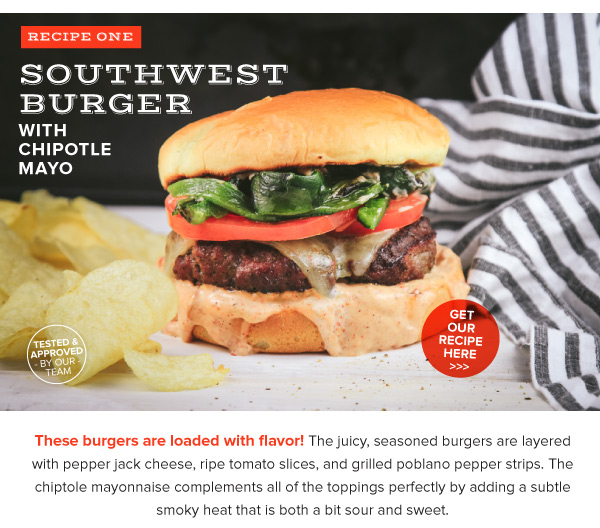Promotional Image for Southwest Burger with Chipotle Mayo Recipe

The image is a promotional graphic for a delectable recipe titled "Southwest Burger with Chipotle Mayo." In the top left corner, a bold red label reads "Recipe 1." Below it, the title "Southwest Burger with Chipotle Mayo" is prominently displayed in striking white text against a solid black background. 

Centrally featured is a mouthwatering burger, showcased on what appears to be a wooden tile or cutting board surface. The burger is composed of a perfectly seasoned beef patty, topped with melted pepper jack cheese, fresh, ripe tomato slices, and grilled poblano pepper strips. The crowning touch is a generous spread of creamy chipotle mayonnaise, enhancing the rich flavors of the burger.

Next to the burger, a handful of crispy potato chips adds a casual, appetizing touch. To the right of the burger, a red circular button invites viewers to "Get Our Recipe Here," accompanied by a round seal that reads "Tested and Approved by Our Team." This seal is accentuated by a descriptive text highlighting the burger's flavor profile: "Loaded with flavor, the juicy seasoned burgers are layered with pepper jack cheese, ripe tomato slices, grilled poblano pepper strips, and chipotle mayo, all topping off with a subtle smoky heat that is both sour and sweet."

Completing the image is a black and white striped cloth napkin partially visible on the right side, contributing a homey and inviting feel to the overall presentation of the recipe advertisement.